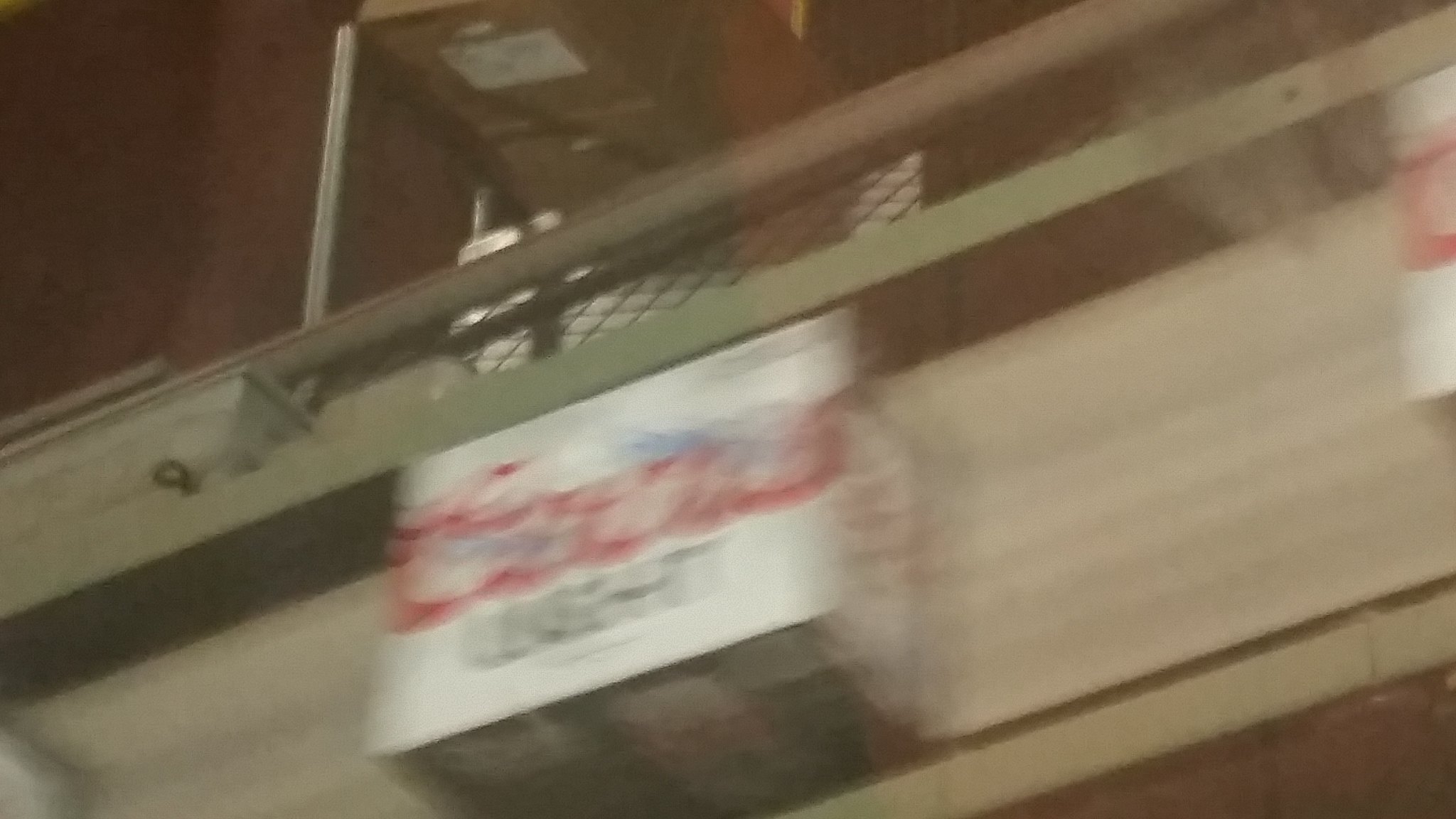The image depicts a slightly blurry view of a conveyor belt system. On the belt, there is a box labeled "Coors Light." The "Coors" logo appears to be in red cursive, while "Light" is black and bold, written in a standard typeface. Although the image quality is poor, you can also make out a small can design on the side of the box. Flanking this box are two additional, similarly labeled Coors Light boxes. The belt itself is beige in color and is supported by a green machine structure. In the background, near the top, there appears to be an additional device and a metal pole on the left. There is also a noticeable black spot in the top left corner of the image.